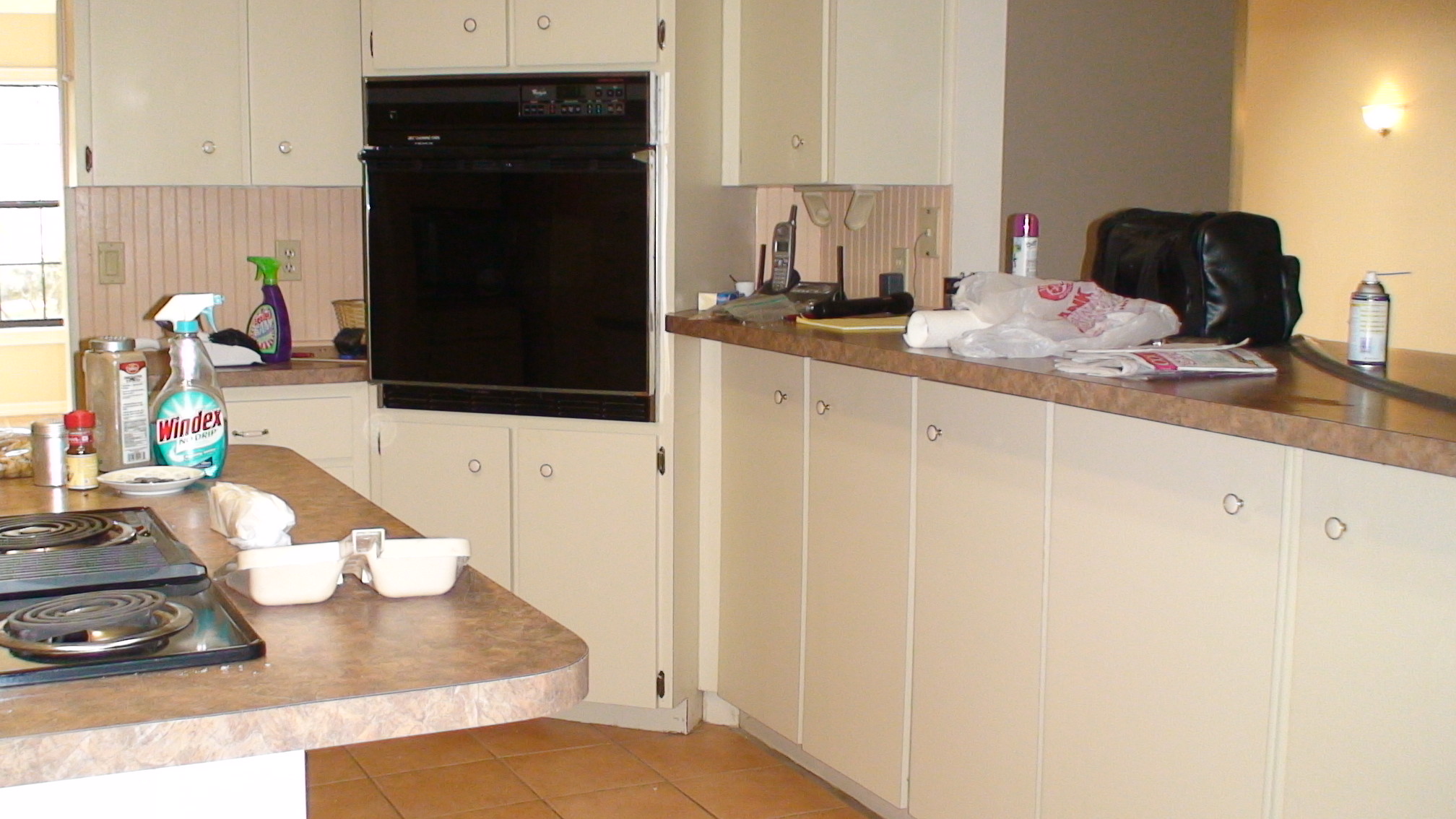The image showcases a well-used kitchen with both upper and lower cream-colored cabinets, providing ample storage space. The floor is covered in dark cream terrazzo tiles with contrasting light grout, adding texture to the room. To the left, a dark-colored countertop houses an embedded stovetop, slightly cluttered with a variety of items including a dust catcher, a bottle of Windex, and several spice jars. A large black oven is built into the far wall among the cabinets, with a cordless phone placed to its right. Nearby, there are spray cans, including a can of WD-40, along with some empty plastic bags and a leather shoulder bag. Additional spray and cleaning bottles are visible to the left of the oven. To the far left of the scene, an opening leads into another room, offering a glimpse of a window and hinting at the home's layout beyond the kitchen.